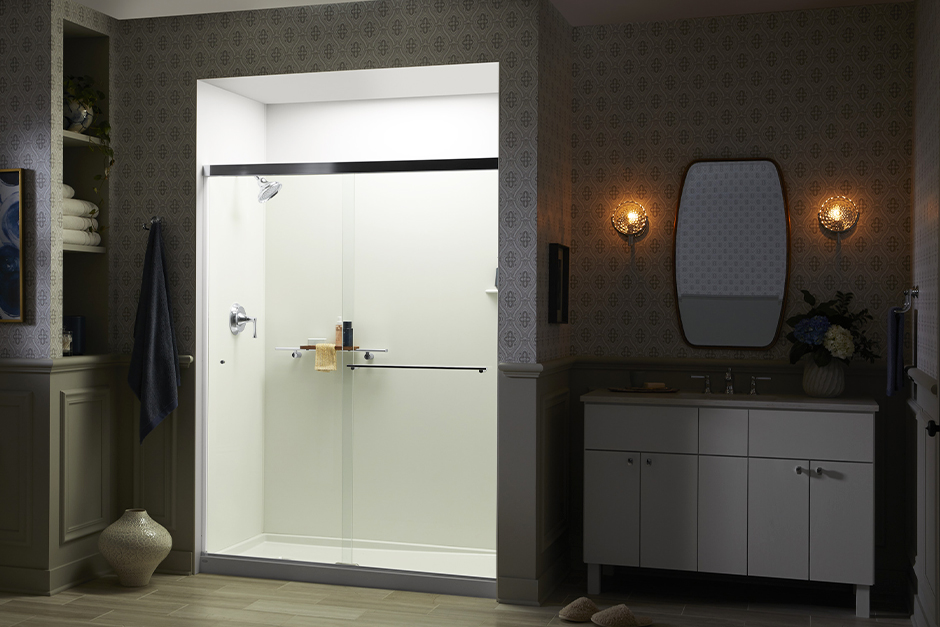The photograph captures an elegant bathroom with a blend of masculine and feminine touches. The lighting is primarily dim, creating a cozy atmosphere, but the shower is brightly illuminated, standing out on the left side of the image. This glass-walled shower features silver fixtures and contains a rag and shampoo. Mounted next to the shower is a blue towel, with additional white towels neatly stacked on built-in shelves. Atop the shelves is a potted plant, enhancing the decor.

To the right, the vanity area includes a single sink set in white cabinets, topped with a soap tray and a flower. A tall mirror is positioned above the sink, flanked by two small sconce lights that provide subtle mood lighting. A hand towel is mounted on the far right-hand wall. The bathroom walls are adorned with greenish-white wallpaper featuring a diamond-shaped pattern that vaguely resembles crosses, adding a refined touch. The floor appears to be a laminate in a beige color, completing the sophisticated look of this bathroom space.